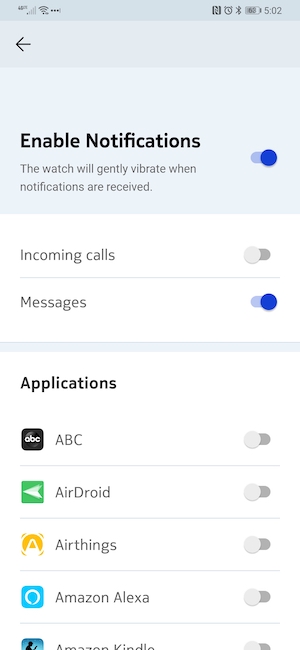The image depicts a smartphone screen displaying the notification settings for a connected smartwatch. At the forefront, the "Enable Notifications" option is prominently featured with bold text, and a light blue highlight box surrounding the description. The option itself is currently disabled, indicated by a greyed-out toggle slider positioned to the left.

Below, an organized section titled "Incoming Calls and Messages" appears, delineated by a blue separator bar. This section is active, as signified by a blue toggle slider switched to the right. Various application notification settings are listed beneath this section. However, all application toggles, including those for "ABC," "AirDroid," "Amazon Alexa," and "Amazon Kindle," are currently disabled, with sliders positioned to the left. Notably, the "Amazon Kindle" entry's logo and name appear partially cut off.

At the top of the screen, the status bar displays essential device information. The time is shown as 5:02, alongside icons indicating a Bluetooth connection and an alarm clock. The signal strength indicators reflect a weak connection, with only one out of five bars for cellular signal and a poor Wi-Fi signal.